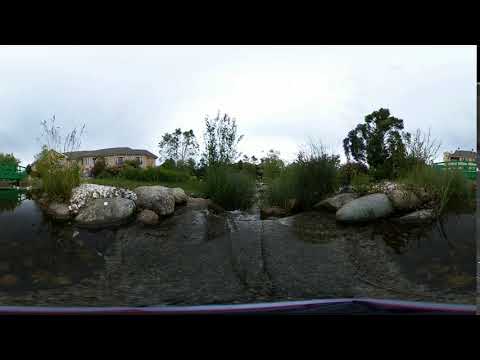This image captures a serene garden pond that appears shallow, situated amongst a meticulously arranged collection of rocks of various sizes and shapes. Framing the scene, at the top and bottom, are black rectangular borders giving the photo a deliberate composition. The foreground is dominated by these decorative rocks, complemented by lush green shrubbery and grass. The water's surface is near the camera’s focus, suggesting a close-up view that envelops the viewer in the tranquil setting.

In the background stands a single-story house with beige siding and a contrasting darker brownish roof. The house is adorned with several windows, contributing to the sense of a picturesque residential garden. The image exudes a calm and overcast ambiance, hinting at a cloudy day, possibly with recent rain, as suggested by the presence of water and the apparent lush greenery. Additionally, the garden is surrounded by verdant trees and bushes, further enhancing the lush and serene environment. This carefully composed shot, with its intricate details of natural and architectural elements, presents a peaceful and inviting garden scene.